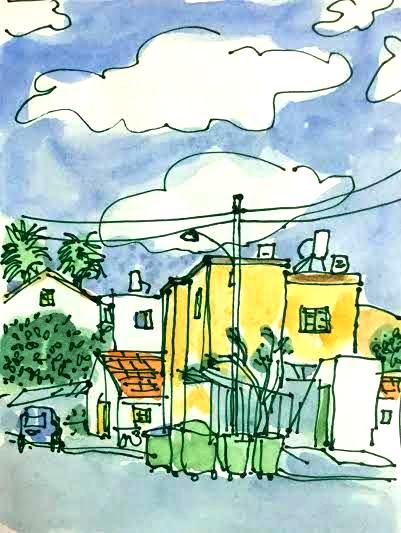The image is a detailed drawing of a city block, enclosed within a rectangular frame where the left and right sides are longer than the top and bottom sides. The top half of the image showcases a vibrant sky, rendered with blue watercolor-like paint, creating a serene background. Within this sky, an array of white, squiggly oval shapes depict floating clouds, adding a dynamic element to the scene.

In the lower part of the image, a gray road runs horizontally, punctuated by a curb lined with multiple trash receptacles. These include two smaller trash cans equipped with circular wheels and a larger green dumpster, also featuring round wheels. Positioned on the left side of the composition, a blue vehicle—potentially a cart or a car—adds a touch of everyday life to the scene.

Opposite the curb and road, a walkway separates the thoroughfare from a series of buildings that line the background. These structures provide an urban context, grounding the scene in the bustling atmosphere of city life.